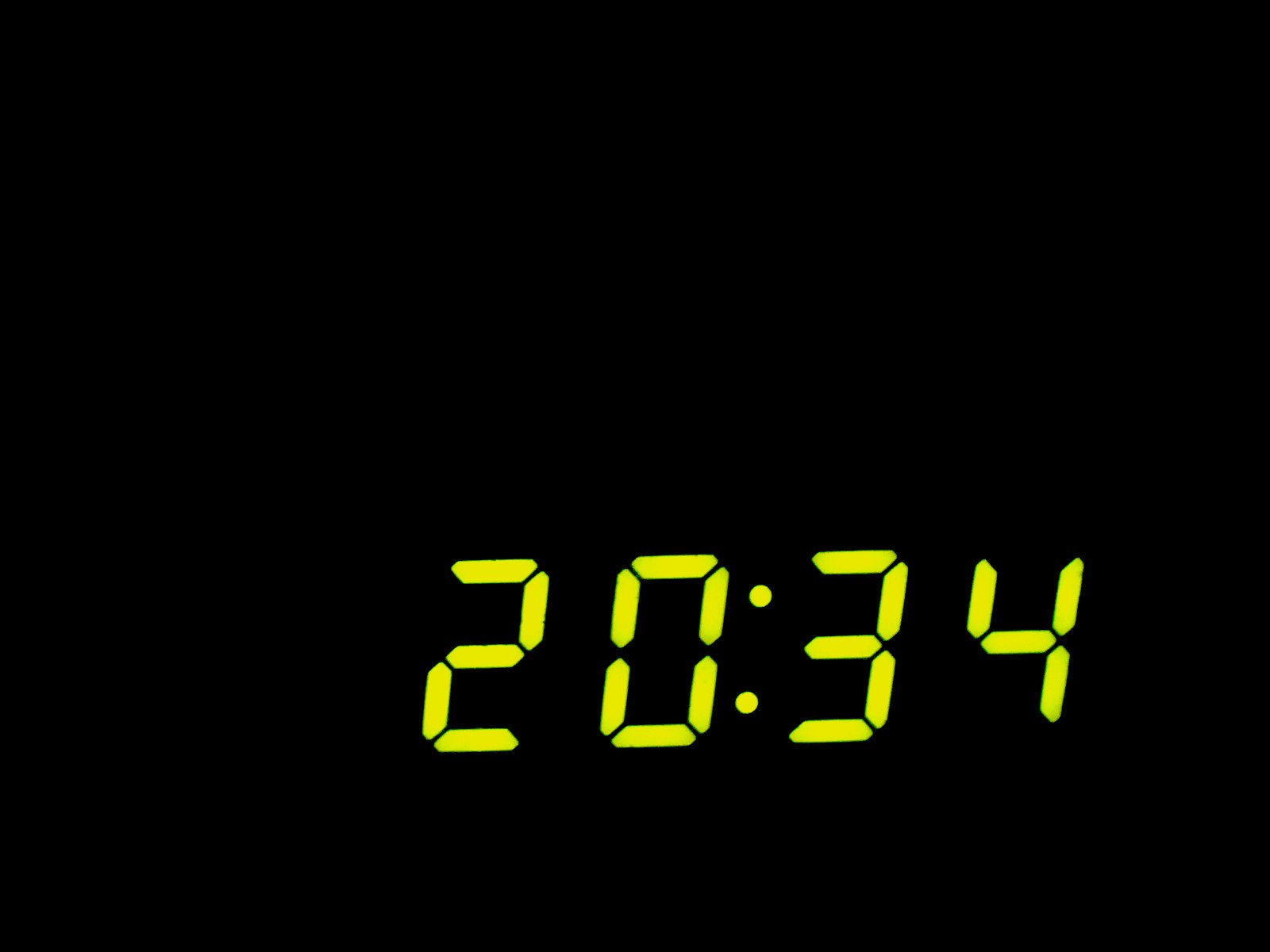In this close-up image, the background is a solid black gradient, filling the entire rectangular frame without any other details or specks of color. Positioned slightly above the bottom left corner and somewhat off-center to the right, there's a digital timestamp that reads "20:34." The numbers are illuminated in a bright yellow hue, which contrasts sharply with the dark background, making them easily readable. The timestamp features distinct numerical formations: the zero, for instance, is crafted from a combination of bright rectangles and lines, with black spaces strategically placed in between. This effect creates a clear and visible display against the black canvas, giving the impression that the numbers could be from a device screen, such as an alarm clock or a darkened cell phone display.